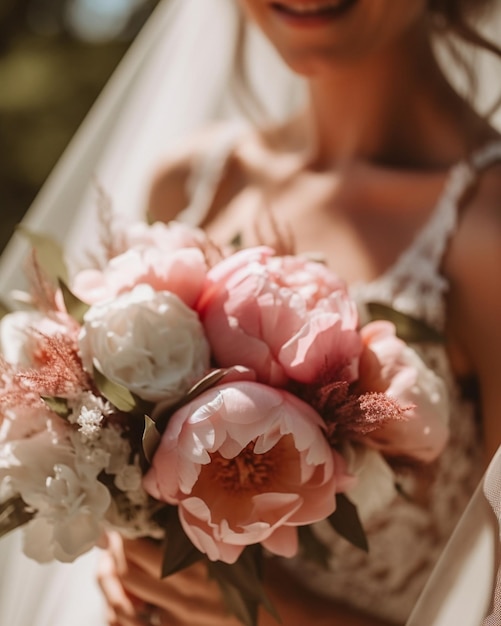This close-up photograph captures a young bride, visible from her smiling mouth down to her torso. She is adorned with a veil draping past her shoulders and is dressed in a white sheer gown with white shawl and straps. Her hands gracefully hold a stunning wedding bouquet positioned at her stomach, featuring a mix of pink and white roses, predominantly with about four big pink flowers and four or five white flowers, interspersed with green leaves and some smaller blooms. The focus is sharply on the bouquet, with the background softly blurred, highlighting the elegance and beauty of the flowers she cherishes.